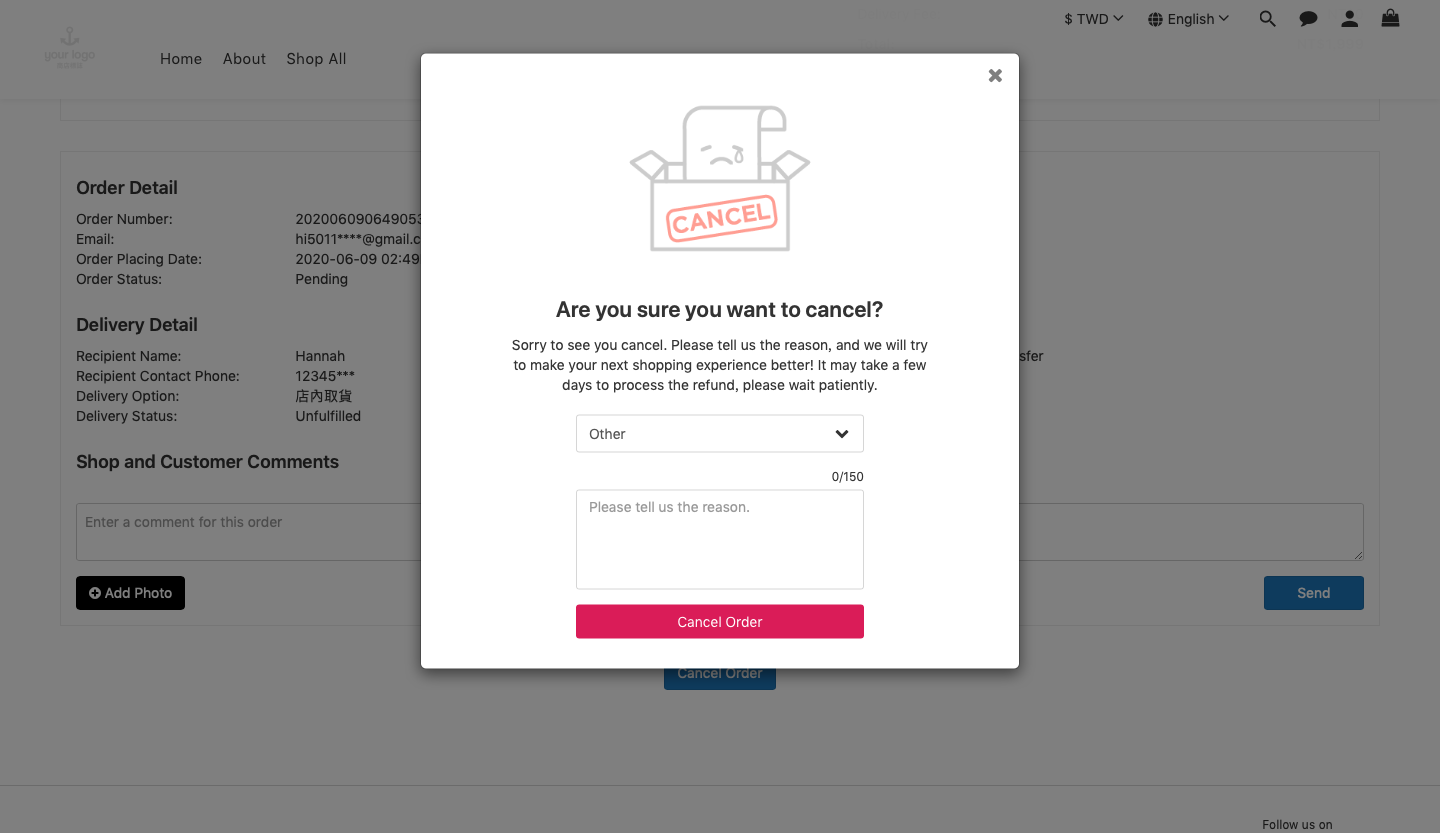The image showcases a computer or laptop screen with various interface elements, highlighting an order cancellation prompt. 

In the background, the website's navigation bar is faintly visible; it includes the options "Home," "About," "Shop," and “All” positioned near the top left, alongside a logo. On the top right, there is a currency indicator displaying a dollar sign followed by "TWD" and an adjacent drop-down menu. To the right of the currency selector, icons for "English" (language selection), a search magnifying glass, a speech bubble for messages, a user profile icon, and a shopping bag are shown.

Delving deeper into the screen's content, visible on the far left are detailed order information records. These details include an order number, an email partially obscured as hi5011******@gmail.com, and the order placement date marked as June 9, 2020, at 2:49 AM. The order status is listed as "Pending." Delivery details are also provided, with the recipient named Hannah and a partially hidden contact number 12345******. The delivery option is described in Chinese and currently marked as "Unfilled."

In the forefront, a prominent cancellation screen is displayed. It features an illustration of a small grey box with a piece of paper protruding from it, depicted with a crying face. The box contains the text "Cancel" in red. A message below asks, "Are you sure you want to cancel?" followed by an apology, "Sorry to see you cancel," and prompts the user to provide a reason for cancellation to improve future shopping experiences. It notes that processing the refund may take a few days and requests patience. The reason selected is marked as "Other," with an option to specify further. Finally, a noticeable pink button at the bottom reads "Cancel Order" in white text.